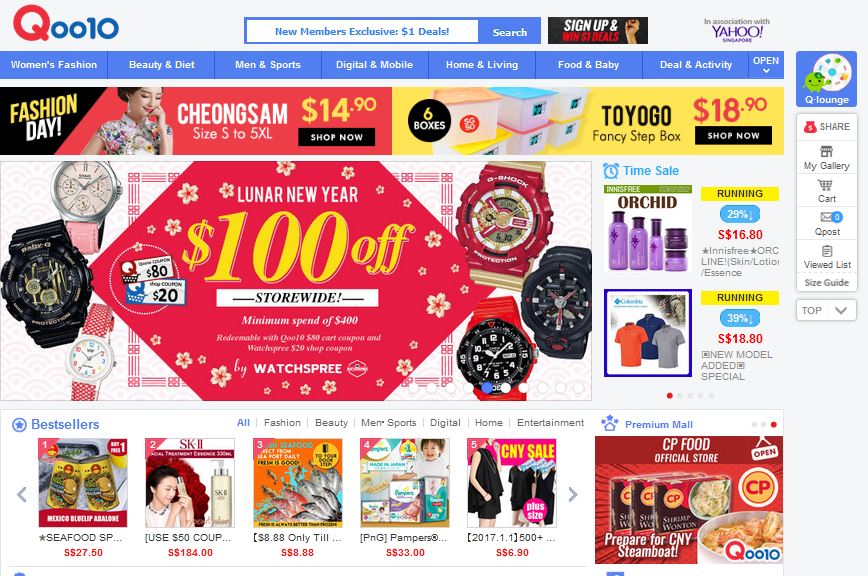**Descriptive Caption:**

Screenshot of an Asian shopping website captured in landscape orientation.

**Top Section:**
- **Top Left Corner:** The website's logo is displayed, consisting of a red "Q" followed by "0010."
- **Top Center:** A blue banner promoting exclusive $1 deals for new members is placed beside a blue search bar. Adjacent to this is a "Sign Up" button.
- **Top Right Corner:** A note mentions that the site operates "in association with Yahoo."

**Right Sidebar:**
- The right-hand sidebar features a section titled "Q Lounge," below which there are options labeled "Share My Gallery," "Chart Q Post," "Notice," "Viewed List," "Size Guide," and "Top."

**Main Navigation Row:**
- Below the top section is a navigation row with a light blue background, displaying categories such as "Women's Fashion," "Beauty and Diet," "Men and Sports Digital," "Mobile," "Home and Living," "Food and Baby," "Deal and Activity." An open down arrow indicates more options are available.

**Main Content Area:**
- The primary content area is filled with numerous images. An Asian woman appears in one of the pictures. Various items with unfamiliar terms like "Cheongsam" and "Toyoga" are displayed, indicating cultural-specific products. There is a reference to "CP Food Official Store" suggesting a variety of Asian food products.

Overall, the website features a diverse range of Asian-themed products and services, including fashion, sports, digital gadgets, home goods, food items, and deals, presented in a visually busy and culturally specific manner.